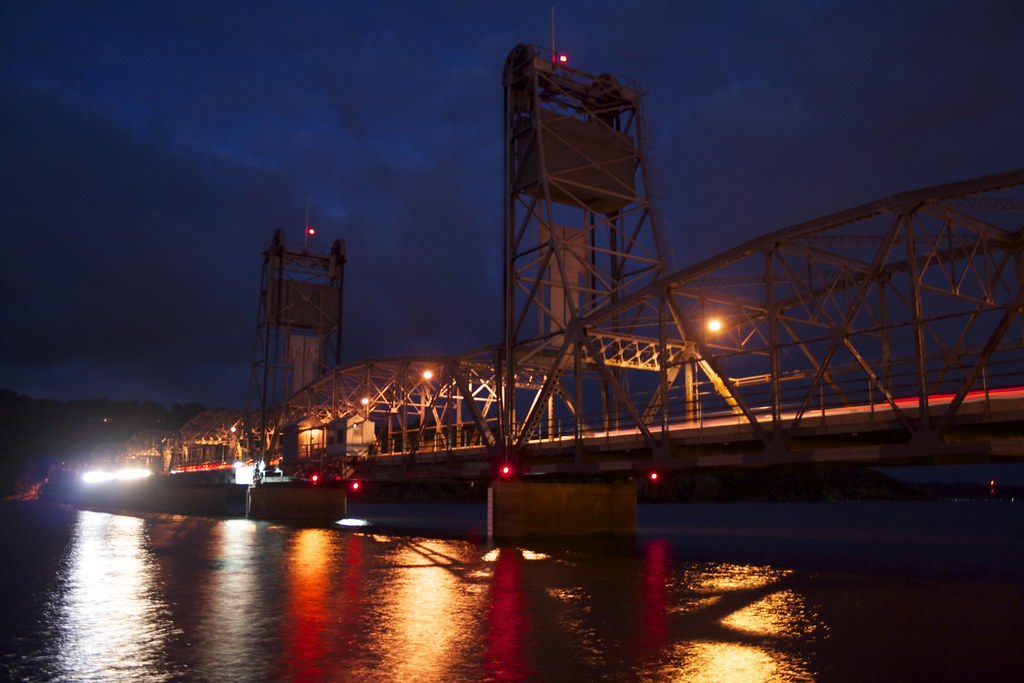The image depicts a photograph of a long, metal bridge extending diagonally from the middle right to the left side of the frame. Dominating the night scene, the bridge is illuminated by numerous bright white lights, especially concentrated on the top overhanging structures and vertical supports. The bridge is built with orange-hued metal, featuring rounded tops and at least three vertical metal supports, two of which are prominently positioned right of center and further to the left in the distance. The structure sits atop solid cement buttresses, clearly visible underneath these vertical supports. Below the bridge, a bluish body of water reflects the myriad lights, creating a serene yet vibrant tableau. The scene also offers glimpses of distant land and hillside under the bridge on the left side. The sky overhead is a rich, deep navy blue adorned with dark clouds, adding to the overall atmospheric elegance of the night setting.